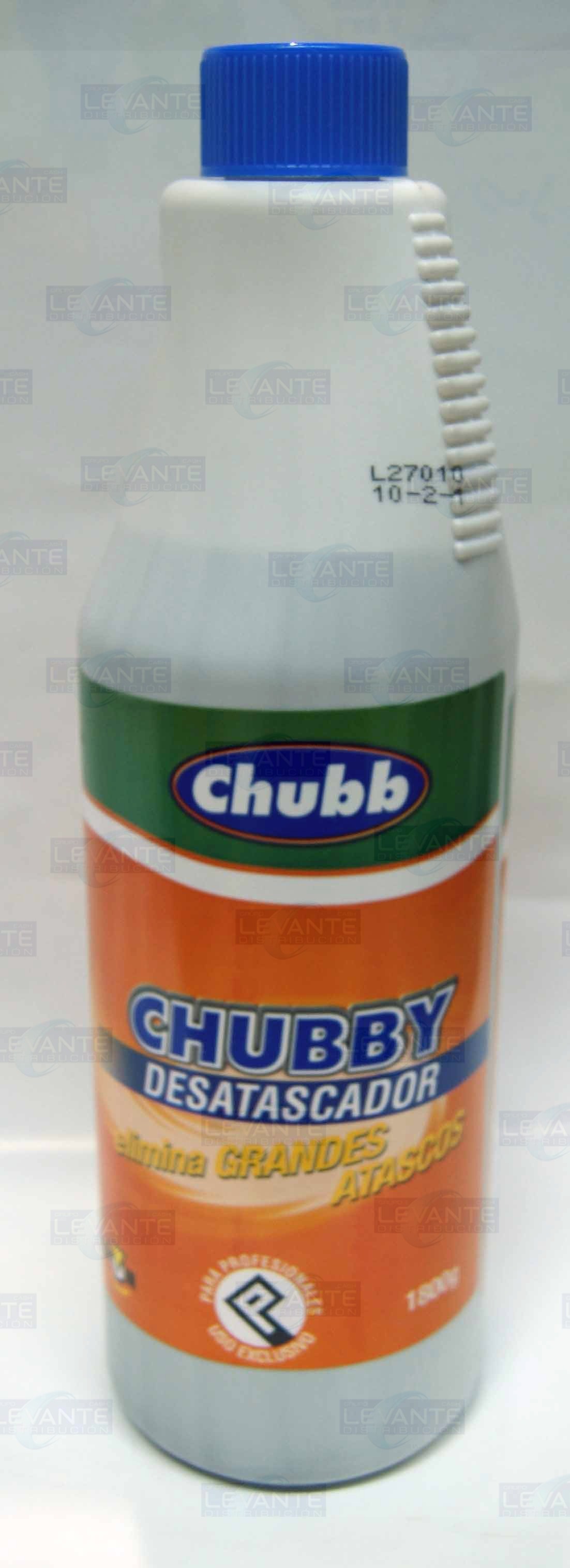This image features a close-up of a distinctive plastic bottle. The bottle is primarily white with a blue cap that has small indentations near the top. Moving down, the bottle transitions to a green color, which could either be a label or the plastic itself. The design includes a blue circle with an orange trim, displaying the word "Chubb" in white letters.

The midsection of the bottle features a prominent orange strip, followed by a large white area and then another significant orange section. In this section, the word "Chubby" is prominently written in blue letters with a white trim. Below this, there is a blue strip with the word "DESATASCADOR" in white letters. Further down, in yellow text, are the words "Elimina Grandes ATASCOS."

At the very bottom of the bottle, there is a white circle with a white 'P' inside a blue 'P'. The bottle sits on a white background, which has a timestamp reading "10-2-1." Above this timestamp, there is a black imprint that reads "L-27010." The background is predominantly white but features faint stamps with the word "Levante" scattered throughout. The purpose or significance of these stamps is unclear.